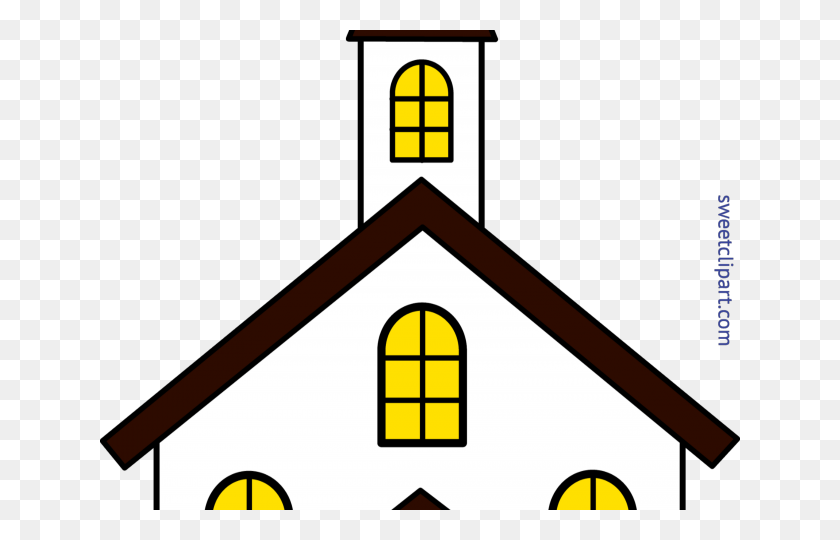This is a detailed clip art image of the upper portion of a house, depicted against a white and purple checkered background. The house features a prominent triangular brown roof with a central chimney extending upward. The chimney, which looks like a white tower, includes an arch-shaped yellow window framed in brown and divided into six panes by a vertical bar, complemented by a thin horizontal brown line representing the top of the chimney. The house itself is white, and below the roof, there is a full arched window with a similar design to the window on the chimney. Flanking the front of the house are two more arch-shaped windows, partly visible, also framed in brown with yellow panes. On the right side of the image, "sweetclipart.com" is written vertically in blue, indicating the source of the clip art.